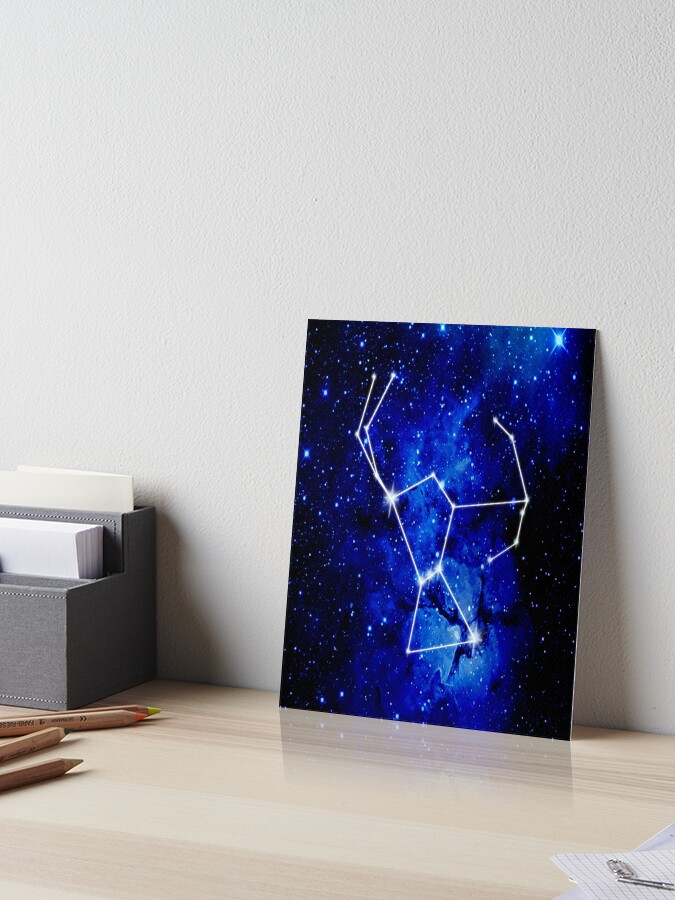The photograph captures a brightly colored print of a constellation, placed at an angle atop a light-colored wooden table in an otherwise empty room. The print, rectangular and vertically oriented, leans against an off-white wall, adding contrast to the neutral tones of the room. Surrounding the print are various stationery items, including pencils, a gray box holding paper and envelopes, and some lined paper alongside a metal key. The print itself depicts a vibrant night sky, featuring a dark expanse filled with stars and a nebula. Amid this starry background, the white outlines of the Sagittarius constellation are prominently displayed, illustrating an archer with a bow and arrow. The constellation is rendered with striking detail, showcasing the brilliance of the stars in bright electric blue against the deep blues and blacks of space.